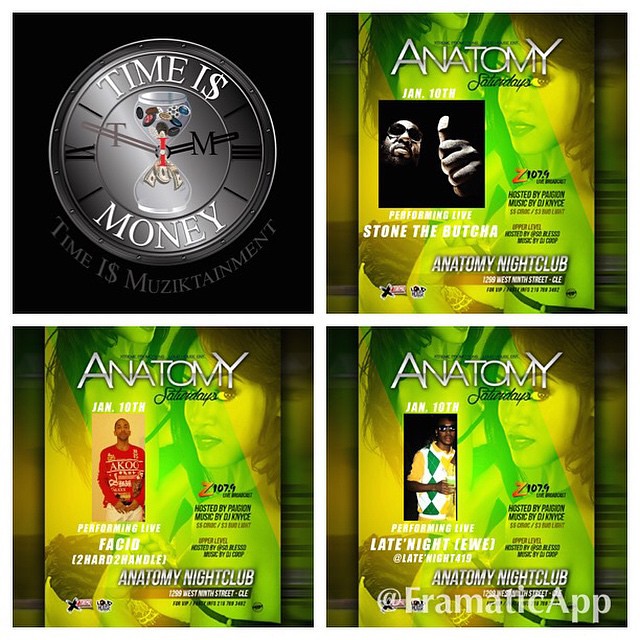This image is a collage of four frames, each serving as an advertisement for an upcoming music festival at Anatomy Nightclub. The top-left frame features a graphic of an hourglass with a clock inside it, adorned with jewelry at the top, and money pouring out the bottom. Accompanying text reads "Time is Money, Time is Music Attainment." The remaining three frames are flyers for the event, each promoting different live performances scheduled for Saturday, January 10th. 

The top-right flyer announces a live performance by "Stone the Butcher," showcasing an image of a Black man wearing sunglasses and giving a thumbs up. The bottom-left flyer advertises "Facet, Too Hard to Handle," with an image of a Black man in a red sweater. The bottom-right flyer promotes "Late Night Yui at 419," displaying a Black man in sunglasses and a green, white, and yellow sweater. 

All flyers include a backdrop featuring a woman with dark hair and are hosted by Z107.9 with music by DJ Nice. Each flyer depicts the Anatomy Nightclub's address, alongside the text "Pragmatic Act." The overall design has a consistent green tint, tying together the individual promotional elements.